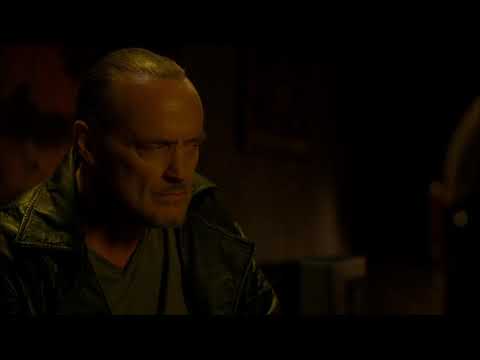This image appears to be a close-up screenshot from a movie or TV show, simulating the look of being on a TV screen with black horizontal strips at the top and bottom. It features an older Caucasian man seated and gazing towards the right. The man has a receding hairline with very short, likely brownish-gray hair, and exhibits pronounced dips under his eyes. He has a small mustache and a bit of a beard, with his mouth closed, giving him a stern or thoughtful expression. He is dressed in a black leather jacket over a dark gray V-neck T-shirt. The background is mostly dark, obscuring detailed elements of the setting, although a blurred wall and a picture can be vaguely discerned. The room appears to be lit from the bottom left, casting shadows that obscure parts of his neck and highlight his facial features.